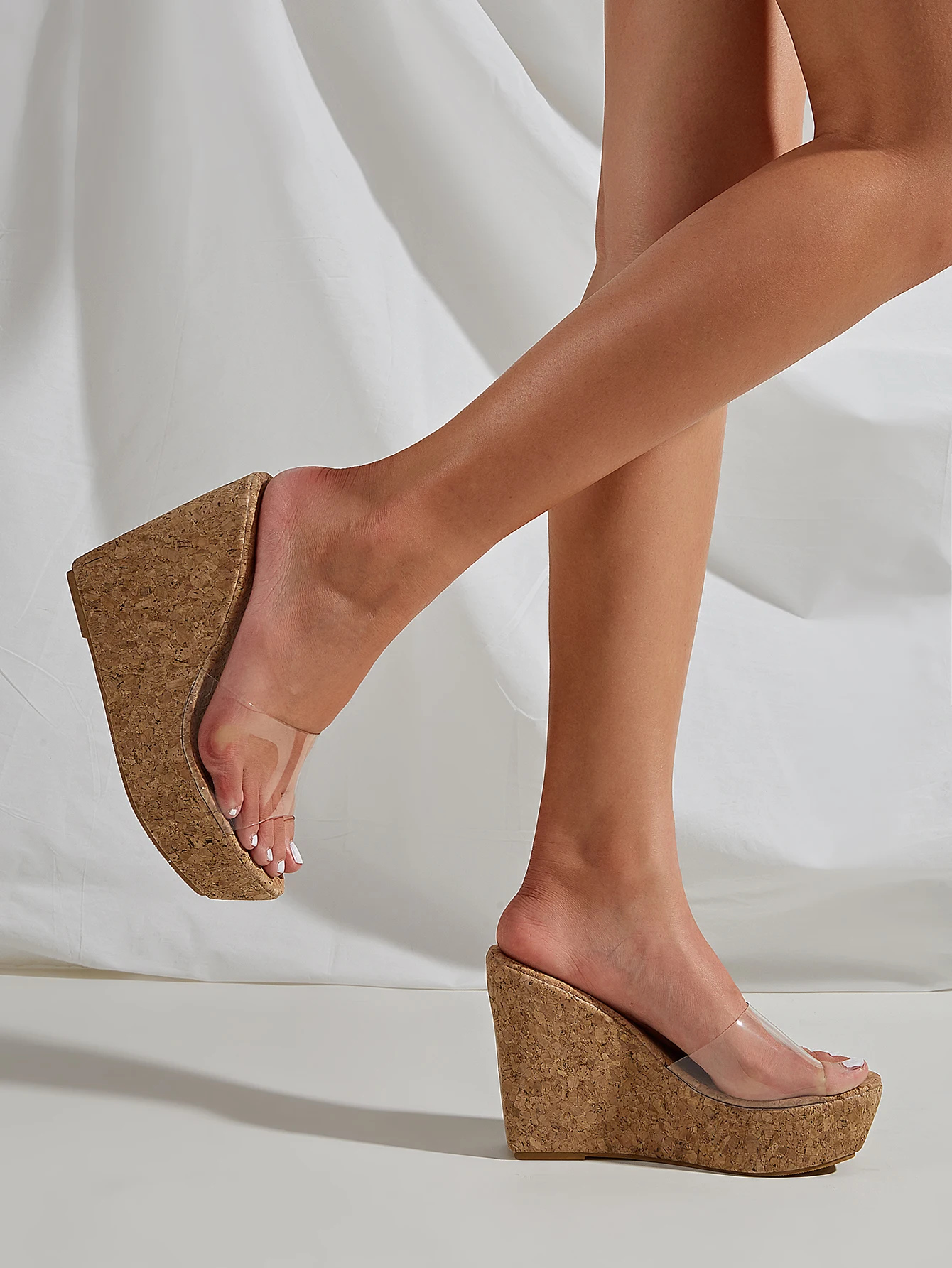This is a detailed portrait-mode photograph featuring a pair of light-skinned female legs from mid-thigh down. The woman appears mid-stride, with her right leg bent at the knee, held up with the foot around six inches off the ground, while her left leg extends straight down, standing on a cream-colored cement floor. She is wearing tall platform sandals with thick cork-like heels that are significantly higher in the back than the front. A clear plastic band secures her feet in the sandals, revealing her white toenail polish. The backdrop of the image, spanning from the top left to the right center, is a dark cream, wavy fabric sheet. Shadows from the shoes extend towards the bottom left, adding depth to the scene. The visible blue veins along the bottom of her left foot add a touch of realism to the composition.